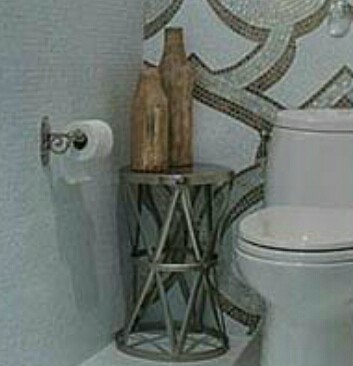The grainy photograph captures a small bathroom scene. Dominating the right side of the image is a white porcelain toilet with both the lid and seat closed. The toilet stands approximately a foot to a foot and a half tall. Just behind and above it, a light gray painted wall serves as the backdrop, partially covered by ceramic tiles in a darker gray, arranged in various directions. The edges of the wall feature an olive green color, adding a contrasting trim to the scene.

In the corner beside the toilet is a dark silver table, nearly matching the height of the toilet. Upon this table sit two brown bottles, likely chosen for decorative purposes. To the left side of the image, the edge of a gray-tiled wall peeks into view, its tiles arranged in small squares. Mounted in the center of this wall is a toilet roll holder with a roll of toilet paper, casting a shadow on the wall behind it. This detailed composition evokes a sense of the intimate and functional nature of the space.